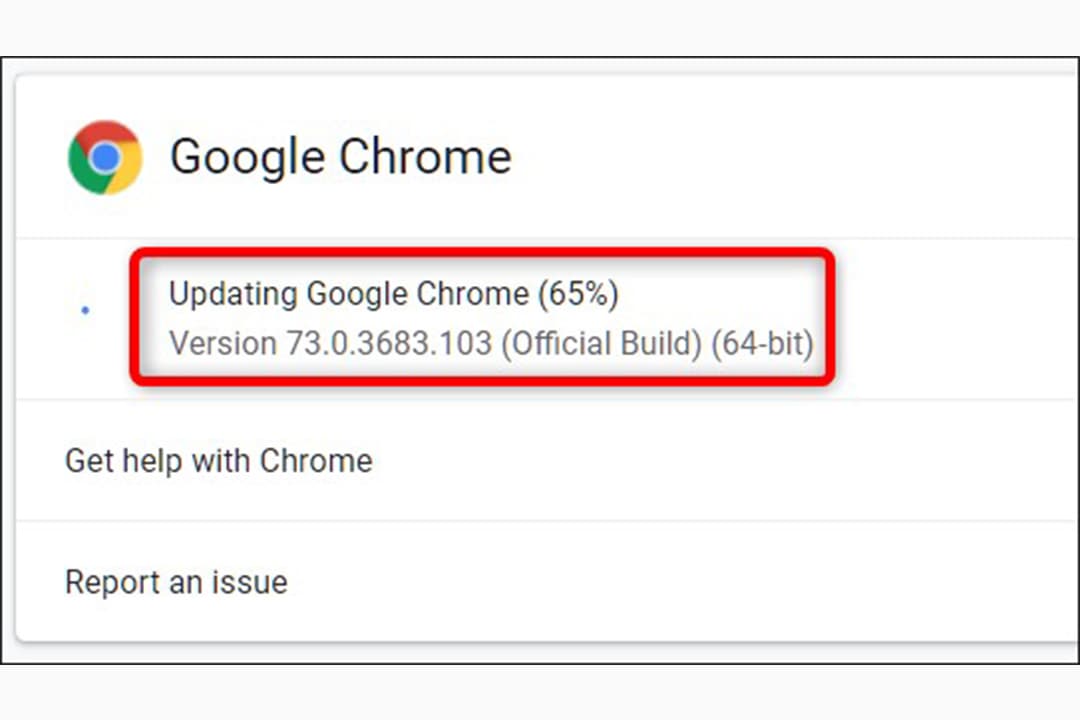A cropped screenshot from the Google Chrome web browser, showcasing a partial view of the update status. At the top, the iconic Google Chrome logo, a circle divided into red, yellow, and green sections with a smaller blue circle at its center, is prominently displayed. Next to the logo, the text "Google Chrome" is visible. The screenshot captures three lines of text, each separated by a faint grey line. The first line, highlighted with a red rectangular box, reads "Updating Google Chrome (65%)" and indicates the progress status. Below it, further details are provided: the version number "73.0.3683.103," labeled as "Official Build," and specified as "64-bit." The second line offers a helpful navigation link: "Get help with Chrome." The third and final line presents an option for users to "Report an issue."